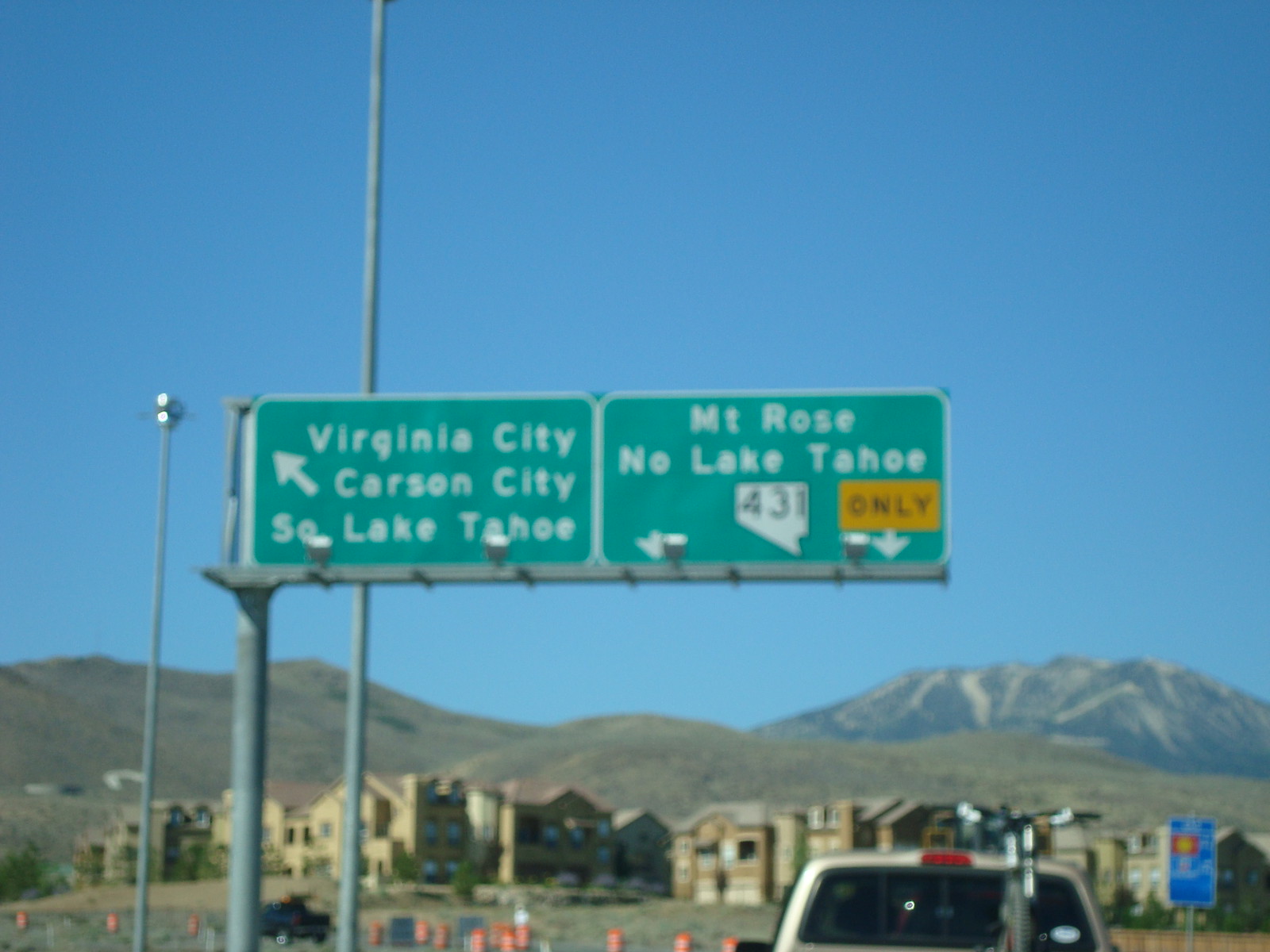The photograph captures a busy highway junction with a prominent road sign on a large metal post located on the left-hand side. The sign consists of two green rectangular panels with white text. The top panel lists destinations: Virginia City, Carson City, and South Lake Tahoe, with an arrow pointing to the upper left-hand corner. The lower panel reads Mount Rose and North Lake Tahoe, featuring the outline of Nevada with the number 431 in black on a white background, and a rectangular sign below that which says 'ONLY' with white arrows pointing downwards on either side.

The scene is set amidst a landscape dominated by a vast blue sky, beige apartment buildings, and a backdrop of rolling hills and mountainous terrain. The mountains to the left display light green grass interspersed with brown and gold patches, while the ones to the right exhibit a mix of dark gray and blue hues, speckled with tan, light gray, and white.

In the foreground, a tan car with a bike mounted on the back is visible, along with orange and white striped cautionary cones scattered along the roadway. A small blue sign is noticeable to the far right. The ground appears barren, devoid of any trees or vegetation. Additional details include a junction indicator where the lanes split: two right lanes lead to Mount Rose and North Lake Tahoe, while the two far left lanes head towards Virginia City, Carson City, and South Lake Tahoe.